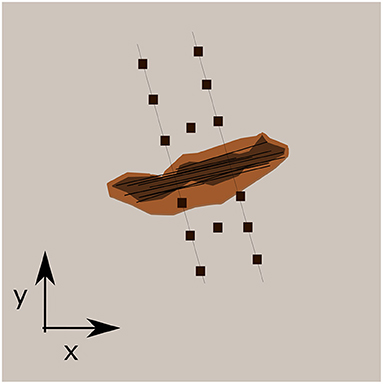The image features an abstract composition with a light peach background. Positioned in the bottom left corner, a set of arrows form an L-shape, with upward and rightward pointing arrows labeled 'Y' and 'X', respectively, suggesting a coordinate plane reference. At the center lies an irregular brown shape, reminiscent of a rock, with a darker brown splotch inside it. This central motif is intersected by two vertically descending lines dotted with black squares, six in total – three at the top and three at the bottom – giving a sense of charting or measurement. Additionally, there are two more black squares one above and one below this brown object, further enhancing the schematic appearance. Lines extend horizontally across the brown shape, adding complexity to the overall design.